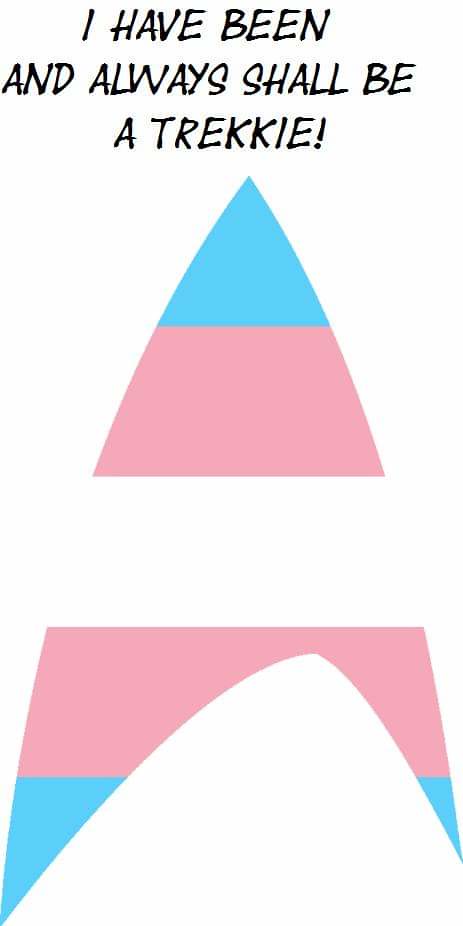The image features a stylized representation of a rocket ship or arrowhead, prominently colored in pink and blue sections. Set against a stark white background, the design is headlined by black, all-capitalized text declaring, "I HAVE BEEN AND ALWAYS SHALL BE A TREKKIE!" At the top of the graphic is a blue triangle, followed by a pink trapezoid. Below this is a white space, succeeded by another pink section, and finally, the design finishes with two blue triangles pointing downwards on either side to form a V-shaped base, giving the entire image a dynamic, spaceship-like appearance. This graphic is possibly designed as a logo or for merchandise, making a bold visual statement about the enduring identity of a "Trekkie."